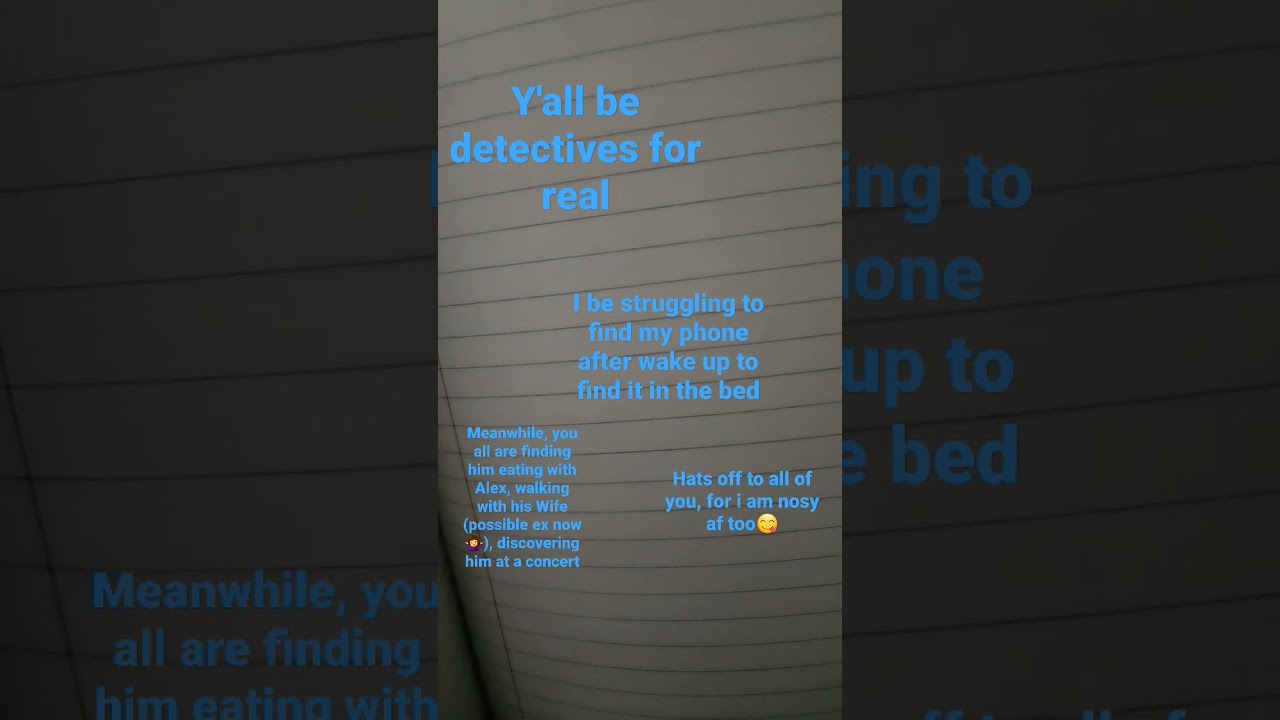The image presents a photograph of what appears to be a piece of lined notebook paper, featuring a slightly tilted view. On the left side, a red vertical margin line runs down the image, accompanied by evenly spaced horizontal lines resembling traditional notebook paper. The background is a light gray, with the horizontal lines in varying darker shades of gray, creating a striped effect. This central image is flanked by dimmed, zoomed-in views of its left and right portions, giving a shaded appearance to the edges.

Situated across the paper in a light blue font, several short, conversational paragraphs are visible. At the top left corner, the text reads, "y'all be detectives for real," written across three lines. In the very center of the image, slightly to the right, another set of text states, "I be struggling to find the path to find it in the dark."

At the bottom left corner, additional text details actions like, "finding him eating with Alex, walking with your wife, possible ex-now discovering you at the concert." Correspondingly, the bottom right corner features the concluding remark, "hats off to all of you, for I am nosy AF too," with a gold smiley face emoji and a tongue-out smiley face emoji adding a playful tone to the message.

Overall, the image narrates a humorous and self-aware commentary on detective-like behaviors in social settings, creatively presented on a visually appealing, notebook-style background.